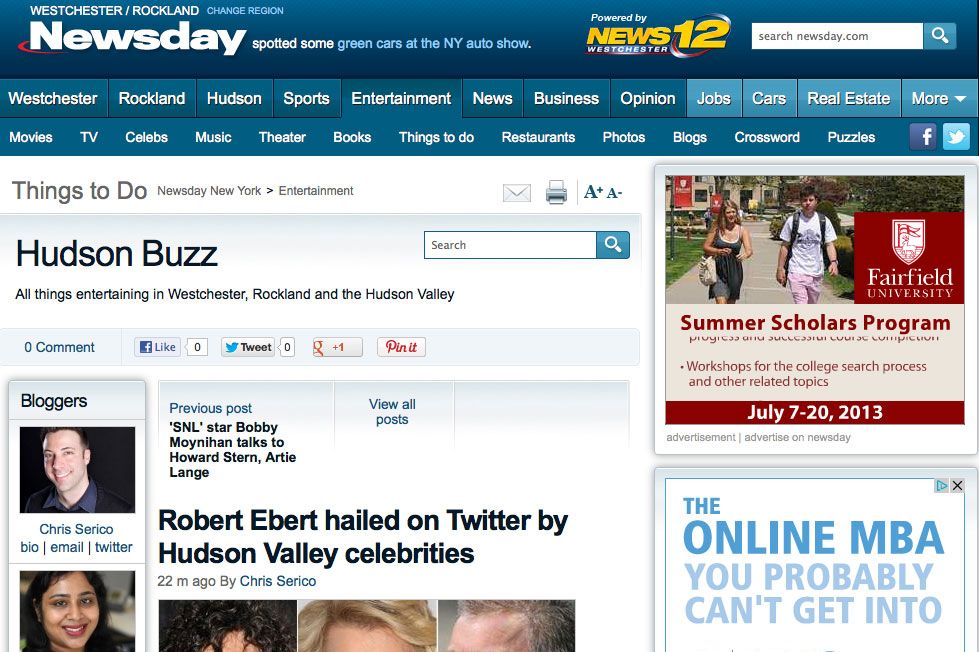This screenshot captures a detailed view of a website interface. At the top left, the website's title "Newsday" is prominently displayed in large, bold white text against a dark blue background. Below this, a lighter blue navigation bar contains menu options in white lettering, including categories like "Sports," "Entertainment," "News," "Business," and "Opinions." To the right, additional buttons for "Jobs," "Cars," and "Real Estate" are similarly styled in white text on a lighter blue background, accompanied by a downward-facing arrow.

Continuing further down, another dark blue menu bar presents more specific sections written in white: "Movies," "TV," "Celebrities," "Music," "Theater," "Books," "Things to Do," "Restaurants," "Photos," "Blogs," and "Puzzles." The main content area below this menu features a white background. The "Things to Do" section is highlighted in medium gray text.

Centered on the page is a headline with the title "Hudson Buzz," likely referencing a city or regional focus, with a subheading indicating coverage of "all things entertaining in Westchester, Rocklin, and the Hudson Valley." Below the headline, an article stands out in bold black text, titled "Robert Ebert Hailed on Twitter by Hudson Valley Celebrities." Further down, the article includes three rectangular photos of these celebrities, although each image is cropped to show only the upper portion of their heads.